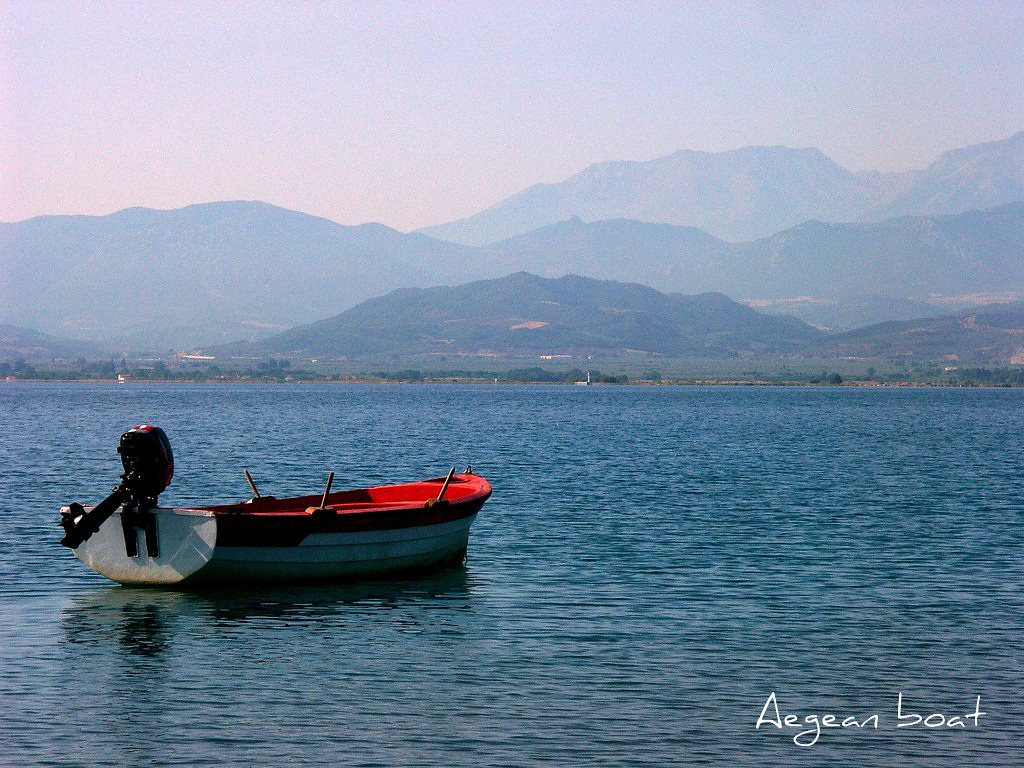The image features a small motorboat with a red interior and white wooden sides, floating vacant on a placid lake with light ripples. The boat, identified as "Aegean Boat" by white text in a handwriting-style font in the bottom right corner, also has wooden handles along its sides and an outboard motor propped upward at the back. The opposite shoreline, approximately a kilometer away, is visible and speckled with trees. Beyond the shore, rows of progressively faded mountains rise up into a mellow sky painted in purplish and reddish hues.